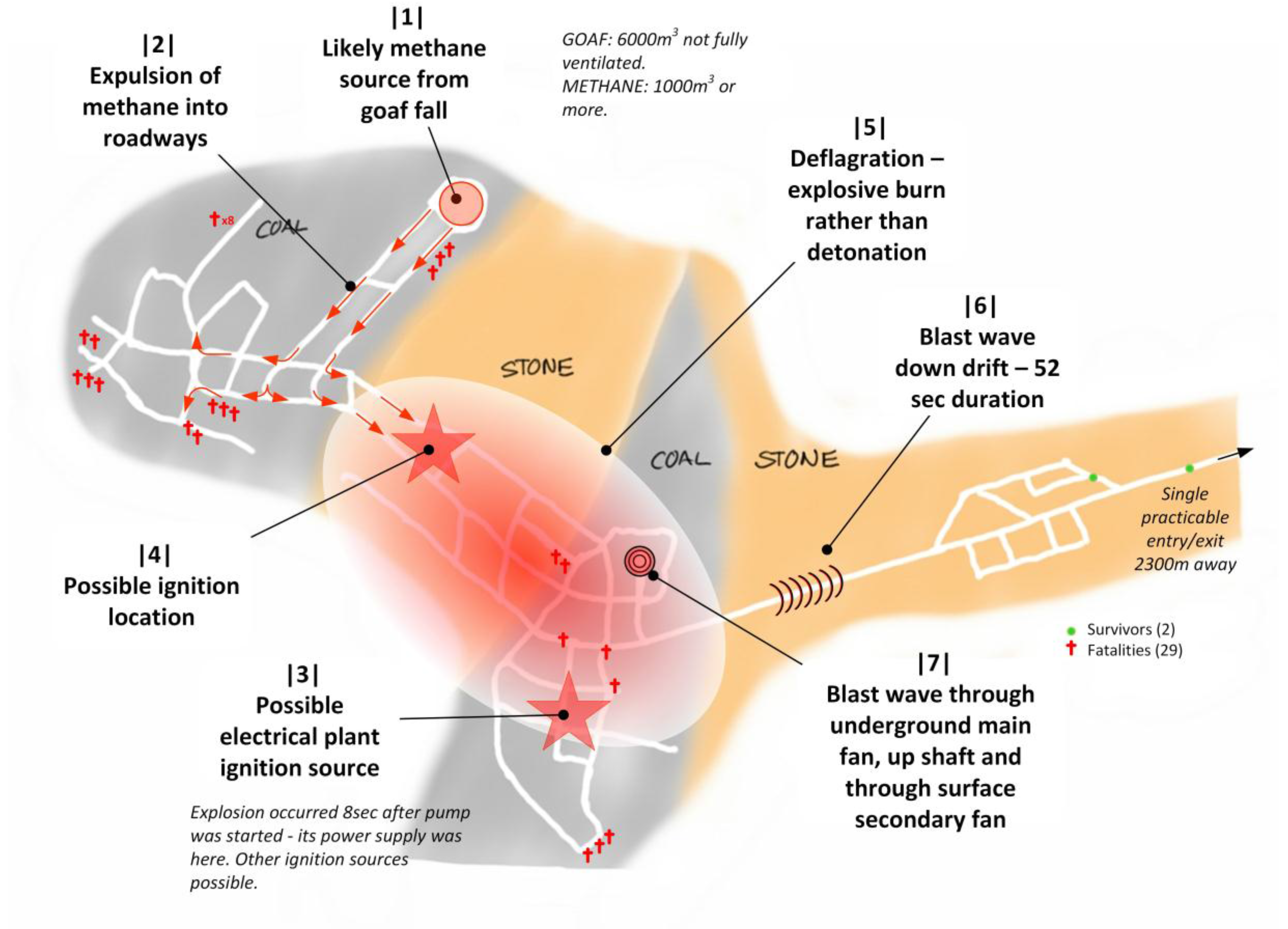This image is a detailed diagram depicting the sequence and possible causes of an underground explosion. It outlines seven key areas: 

1. Likely methane source from a goaf fall.
2. Expulsion of methane into the roadways.
3. Possible electrical plant ignition source.
4. Potential ignition location.
5. Deflagration, indicating an explosive burn rather than a detonation.
6. Blast wave down drift with a 52-second duration.
7. Blast wave through the underground main fan, up the shaft, and through the surface secondary fan.

The image includes symbols and labels such as a tangle of white lines at the top left corner signifying the explosion of methane, and other elements colored orange and gray denoting stone and coal. The diagram also tragically notes the aftermath, indicating 2 survivors and 29 fatalities, aiming to analyze the causes and mechanisms of the blast to prevent future incidents.